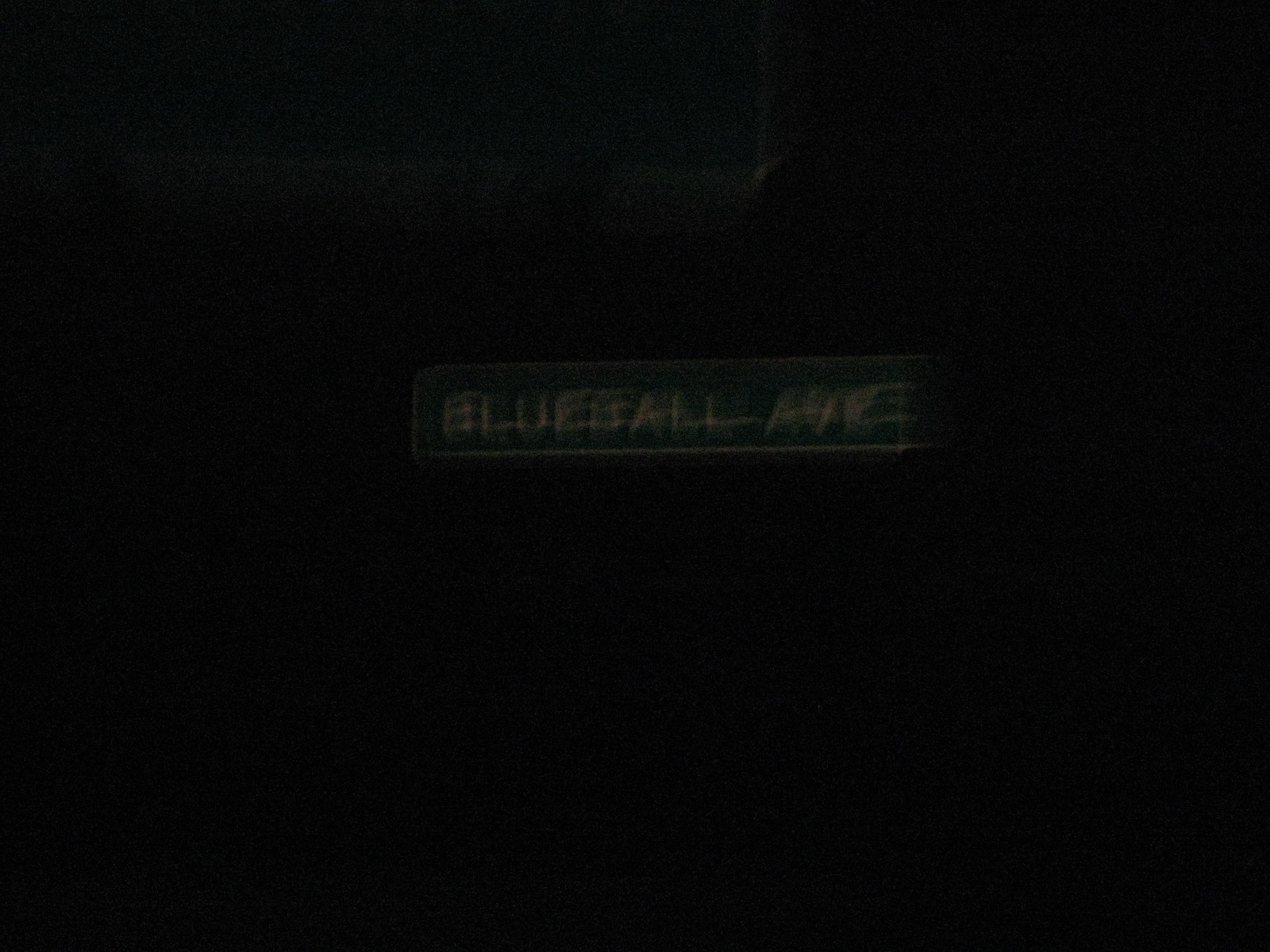A green sign with a white border prominently displays the text "Blue Ball Avenue" in white lettering against a completely black background. The surrounding area is engulfed in deep darkness, obscuring any other visible elements. Below the sign, there is a slightly blurred action shot, likely captured from a moving camera, adding a dynamic sense of motion and contrast to the otherwise stark and static scene.